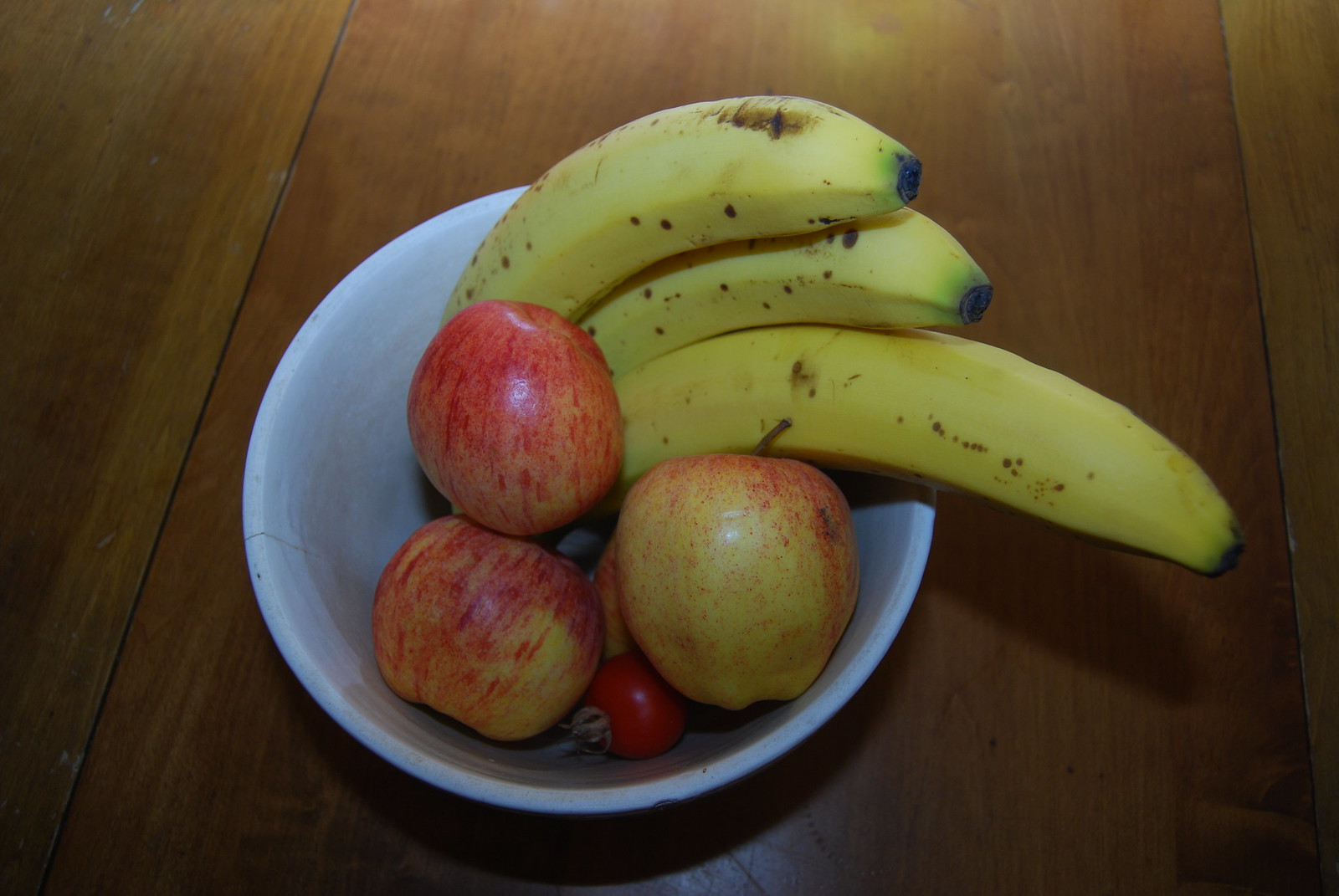A vibrant bowl of fruit is set against the backdrop of a rustic brown wooden table, its fibers running vertically and subtly shaded with hints of gray towards the bottom right and left, gradually brightening towards the top center where light cascades down. Within the bowl, three yellow bananas are arranged with two of similar length lying side by side, while a longer third banana slightly protrudes. The bananas are speckled with brown spots, displaying a faint green tinge near the tips, blending into black on the ends. Accompanying the bananas are three apples, their red skins adorned with vertical yellow streaks. The largest apple is positioned on the right, while a medium-sized apple rests at the bottom left and the smallest one is placed at the top. Nestled among the fruits is a single cherry tomato with its stem upright, adding a pop of vibrant red to the ensemble.